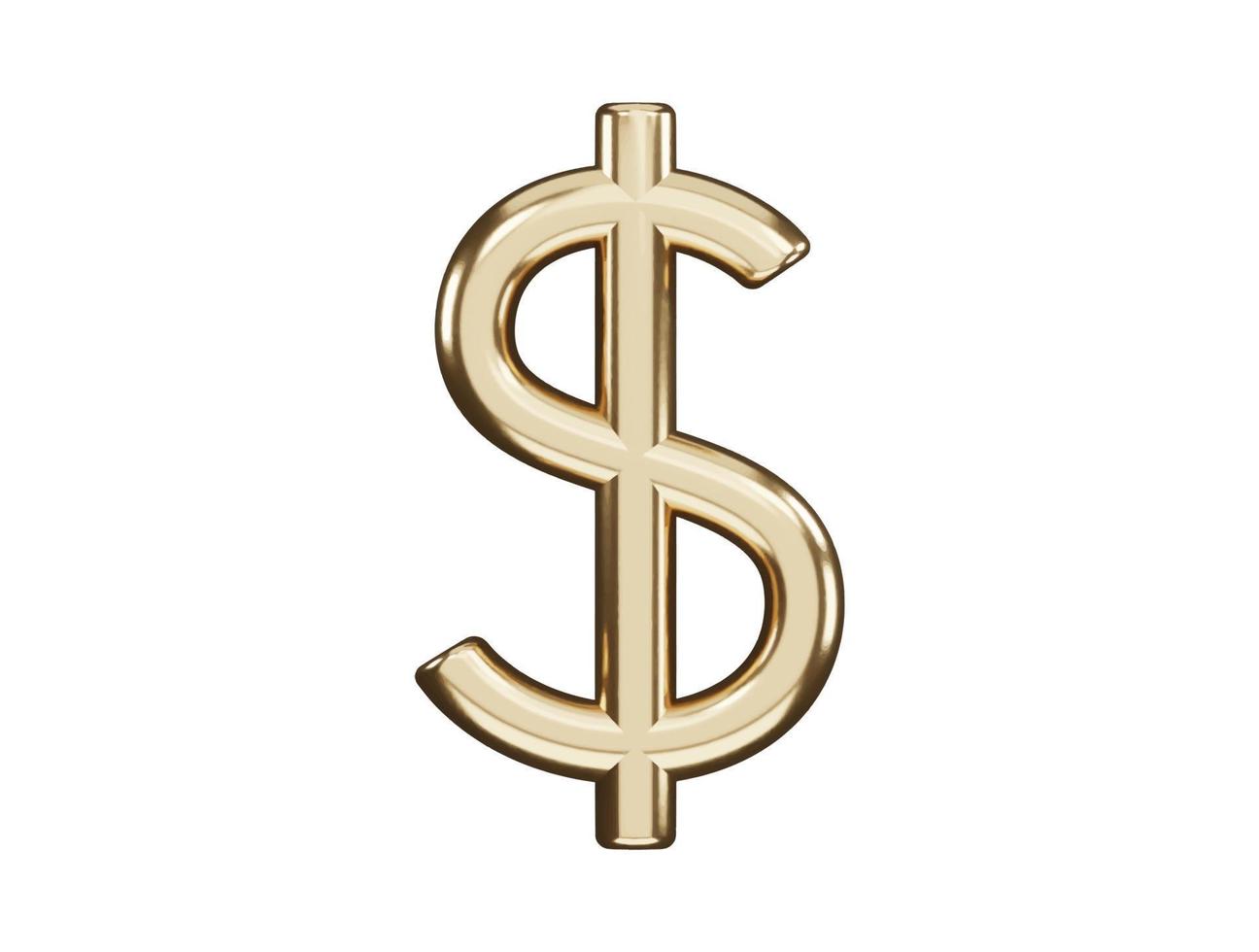This is a photo of a shiny metal dollar sign that appears to be crafted from gold or brass. The dollar sign features an 'S' shape with a bar running vertically through its center. It is set against a white background, emphasizing its metallic sheen. The object seems versatile; it could be perceived as a brooch, given the presence of a pin on both the front and back sides, or as a component potentially used in construction due to its robust appearance.